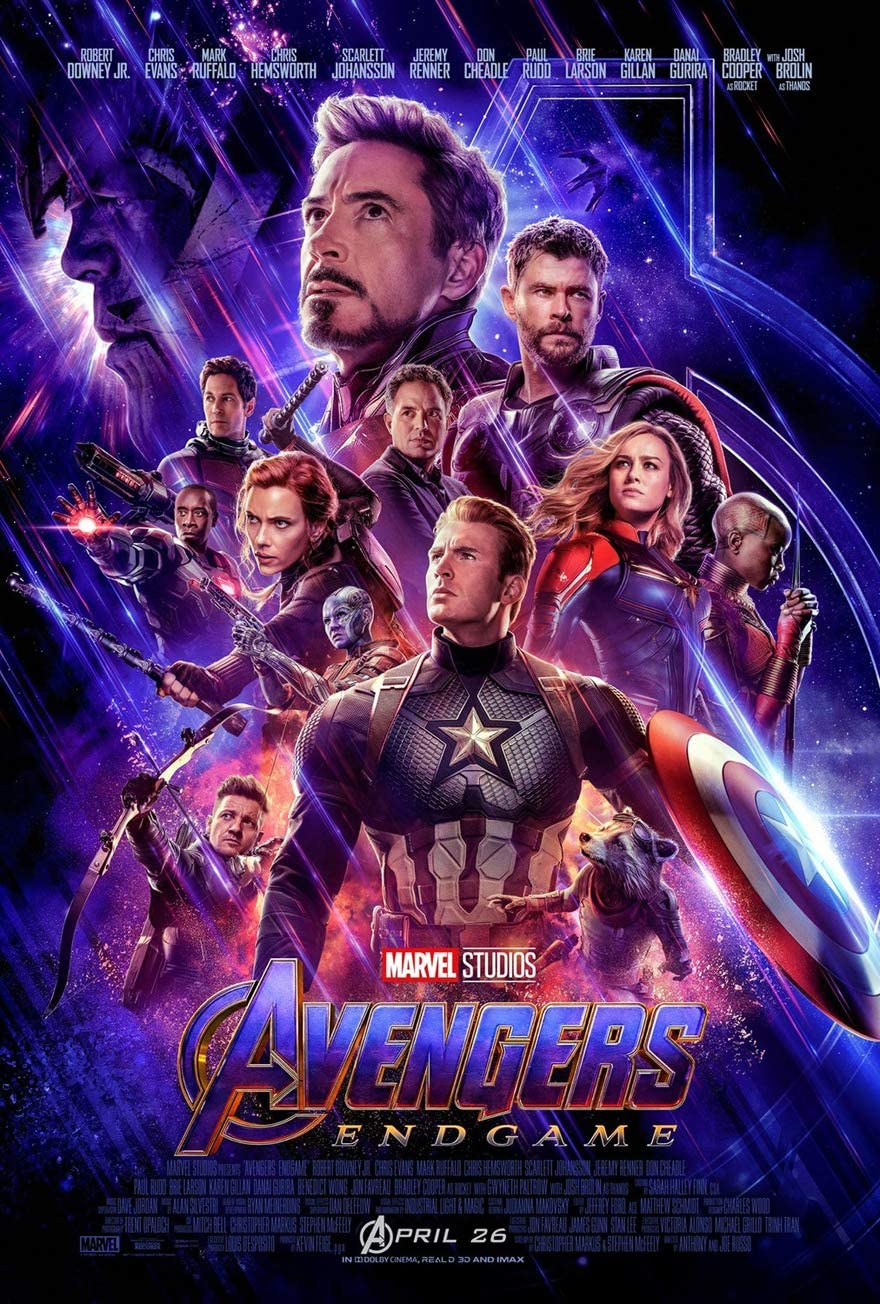The movie poster for "Avengers Endgame" features a predominantly black background with accents of light blue and purple lighting. Across the top, the names of approximately 12 actors are displayed in small white text. The central figure is Captain America, positioned chest-forward, with his head slightly tilted up and to the left. He holds his iconic red, white, and blue shield on his left arm. Below his waist, in a red box with white lettering, is the Marvel logo, followed by "Studios." Beneath this, in large blue letters, it reads "Avengers," with "Endgame" in white lettering directly underneath.

To the left of Captain America is Hawkeye, depicted mid-shot with his bow and arrow. Underneath Captain America's arm is Rocket Raccoon, facing the camera. Surrounding these central figures are several other heroes and characters from the Marvel universe. Notably, Black Widow is positioned above Hawkeye, with Gamora slightly below her. Rhodes, poised to shoot a beam from his hand, is to the left of Black Widow, and above him is Ant-Man. 

Prominent in the upper section of the poster is Tony Stark (Robert Downey Jr.), looking upwards with a serious expression. To his right is Bruce Banner (Mark Ruffalo), and next to them is Thor (Chris Hemsworth), wearing armor and wielding his hammer. Captain Marvel (Brie Larson) is placed below Thor, with one of T'Challa’s warriors to her left, holding a spear.

Additionally, Thanos' head can be seen in the background on the left side of the poster, rendered in purple and black, slightly tilted downward and leftward. At the bottom of the poster, aside from the movie's title, there is also a small text that reads "April 26th." The various characters are framed by the striking blue and purple hues, making them stand out against the dark background, while the mix of male and female heroes highlights the ensemble cast within the Avengers lineup.